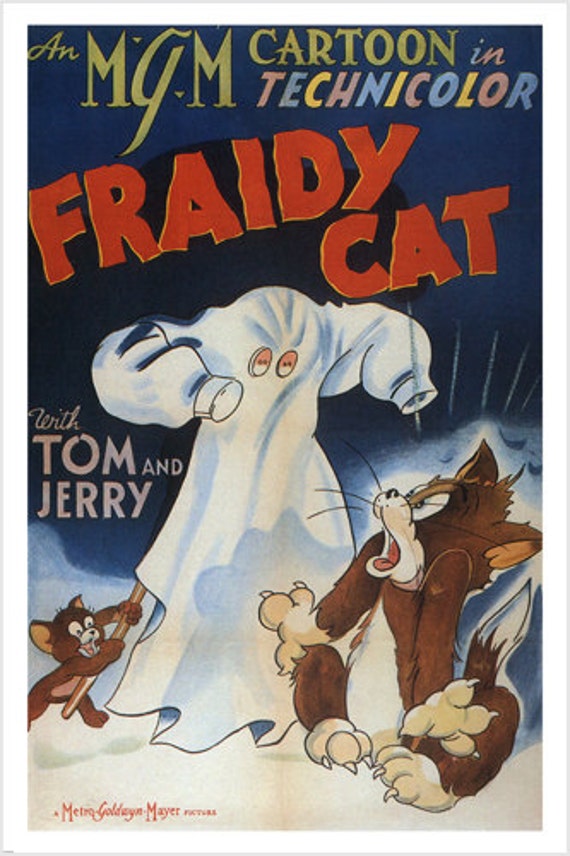The image is a colorful, vintage-looking cartoon poster resembling the cover of an old VHS tape for a Tom and Jerry episode. At the top in yellow, it says "An MGM Cartoon," followed by "in Technicolor" in multicolored italics of pinks, blues, and yellows. The title "Frady Cat" is prominently displayed in bright red, bold letters with a gold outline. The background is a gradient of dark blue to black, suggesting a nighttime scene possibly set in the snow.

Central to the image, a ghostly figure with button eyes and sleeved hands looms, but it's an illusion created by Jerry the mouse, who is holding up the ghost with a wooden skewer or pole. Jerry is positioned at the bottom left, gleefully laughing, while Tom, the cat, is on the right side, petrified, with his mouth wide open, shaking, and claws extended. The bottom left corner of the image includes the text "Metro Goldwyn Mayer Pictures." This vibrant, nostalgic poster effectively captures the classic and mischievous spirit of the Tom and Jerry cartoons.